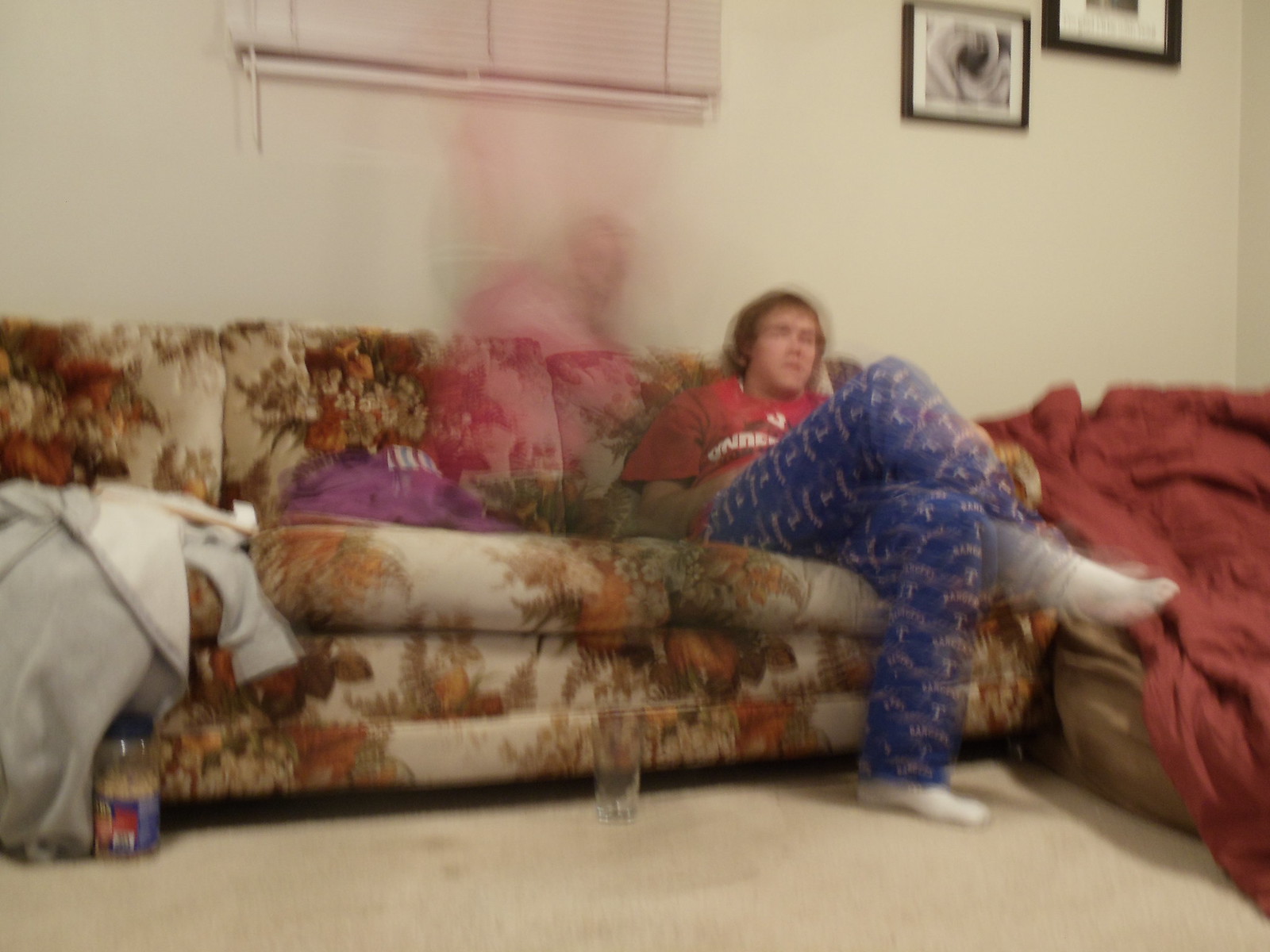In the provided image, although distorted and blurry, an individual can be seen seated on a floral-patterned couch with their legs crossed. The person is dressed in a red shirt, blue pants, and white socks. Adjacent to them, an extremely faint and almost transparent figure of another person is barely visible, adding to the mystique of the scene. On the floor in front of the couch, there are a jar of peanuts and a glass cup, suggesting a relaxed, casual setting. The right side of the couch is partially draped with a red blanket, adding a touch of coziness. In the background, a white wall adorned with picture frames and a window shade can be observed. Despite the significant blurriness and distortion, the image is brightly lit, bringing an overall sense of warmth to the scene.